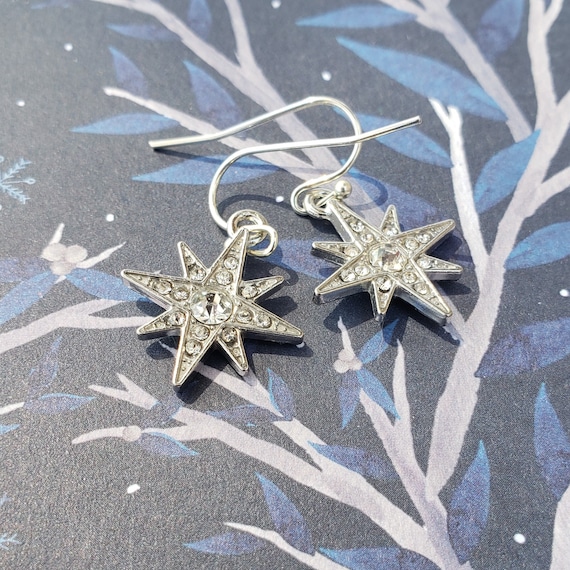The photograph displays a pair of silver, star-shaped earrings placed on what appears to be a black surface adorned with a textured print reminiscent of tree branches with leaves. These branches and leaves are depicted in shades of white, dark gray, and dark blue, with additional small white dots scattered around, resembling stars or possibly snowflakes, creating a sense of a winter night. The earrings are positioned centrally within the frame and feature a prominent clear jewel at the center. Each of the six large triangular points of the star holds an additional jewel, with the largest nearer to the center and smaller ones towards the tips. Additionally, each of the smaller triangles radiating diagonally from the center also contains a jewel. The earrings are equipped with large, thin hooks for wearing, completing their intricate and elegant design.